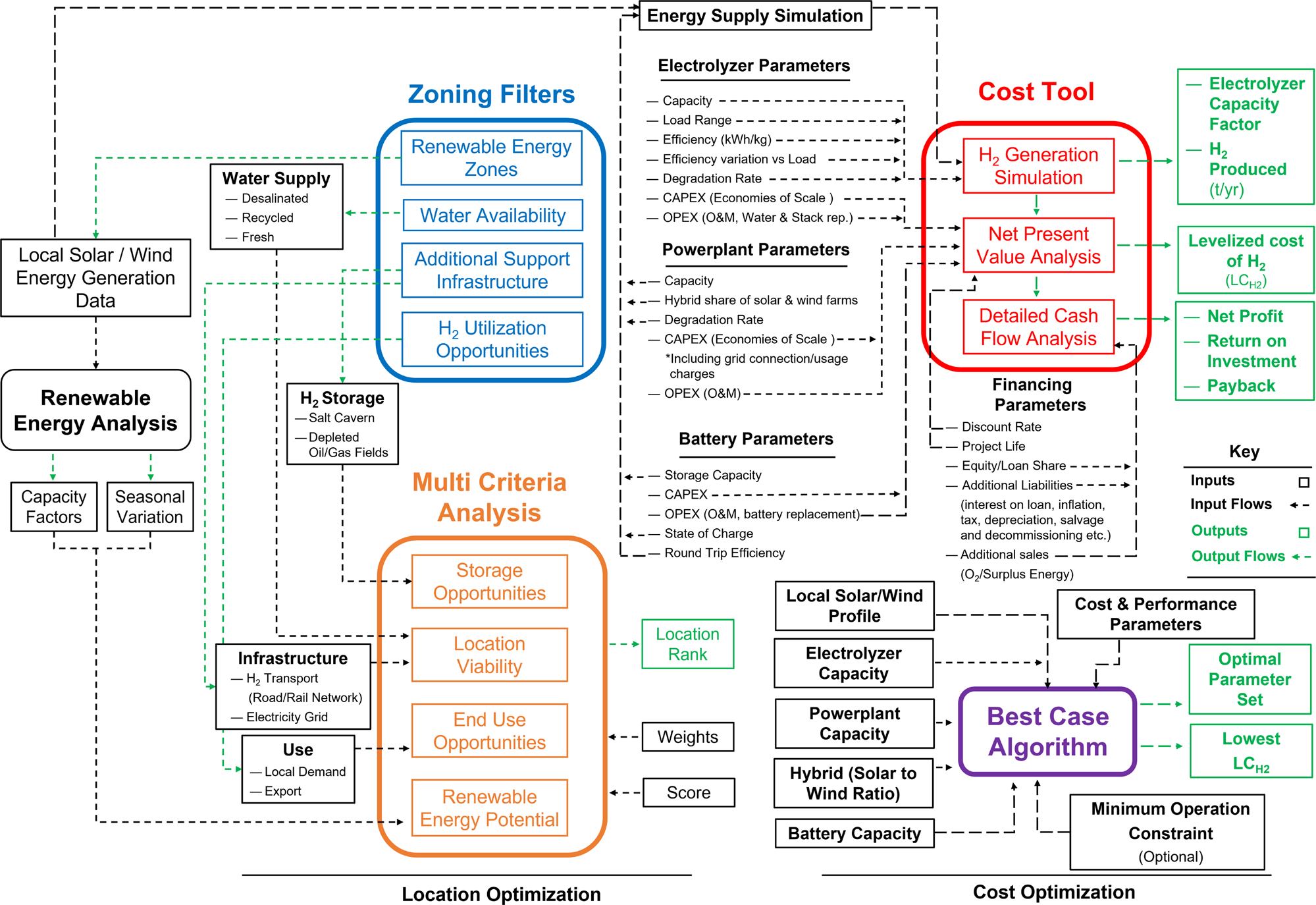The image is a detailed and complex printout of an energy supply simulation. It is labeled "Energy Supply Simulation" at the top and is divided into multiple sections, each highlighted with specific colors such as green, orange, purple, blue, and red. On the left side, it focuses on "Renewable Energy Analysis," which includes data on local solar and wind energy generation, and is outlined in black. This section feeds into "Zoning Filters," considering renewable energy zones, water availability, and multi-criteria analysis, which is marked in orange and includes factors like location viability and end-use opportunities.

In the middle, black text details parameters relevant to electrolyzers, power plants, and batteries. The bottom right side discusses the "Best-Case Algorithm," shown in purple, which incorporates local solar and wind data, battery capacity, cost and performance parameters, and minimum operation constraints. The top right section is dedicated to the "Cost Tool," addressing the financial aspects of the simulation, including cost optimization and net profit. This intricate chart also features a key that delineates inputs, input flows, outputs, and output flows, emphasizing its comprehensive nature.